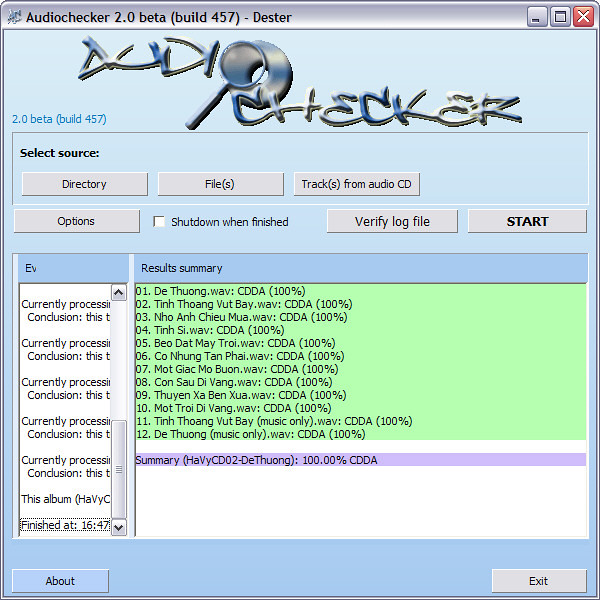The image depicts a computer log screen from an old-fashioned operating system, likely Windows 2000 or Windows XP, showcasing the application "AudioChecker 2.0 Beta Build 457-Duster." The window has a gray border thickest at the top, with standard minimize, maximize, and close buttons in the top right corner. In the top left, the application title and build number are written. Centrally, the logo "AudioChecker" is displayed in a metallic font with a magnifying glass as the 'O'. Beneath this logo, the instructions prompt to "Select Source," offering options such as directory, files, or tracks from an audio CD. Accompanying buttons include options, shutdown when finished, verify log file, and start. The lower half of the screen features a "Result Summary," listing 12 songs on a green background in black font, and a purple rectangle below reading "Summary." The summary line indicates "100% CD da" with file types mainly being .wav. The entire layout is designed to look like a page from an older computer system detailing the steps and results of an audio check process.